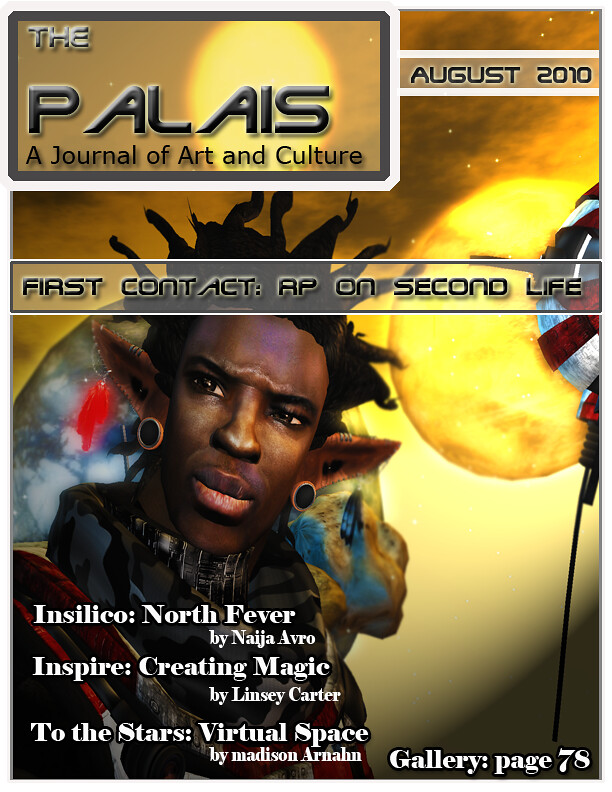The cover of the August 2010 issue of *The Palais: The Journal of Art and Culture* showcases a sci-fi themed design. The title, rendered in a futuristic font, is prominently displayed at the top left, with the issue date to the right. The main feature, "First Contact: AP on Second Life," is clearly highlighted. Dominating the cover is a 3D rendering of a black man with short dreadlocks, pronounced elf-like ears, large plug earrings, and spiky hair. He is dressed in distinctive high-colored attire that resembles a black, red, and white spacesuit or armor. The graphical style, slightly dated, suggests an early 2000s aesthetic. The character is set against a vibrant yellow background, featuring a glowing planet or sun, a larger blue planet, and a spaceship or satellite amid a nebula. Additional article titles include "Insilico North Fever" by Nadja Avro, "Inspire: Creating Magic" by Lindsey Carter, and "To the Stars: Virtual Space" by Madison Arula, with a mention of a gallery on page 78.